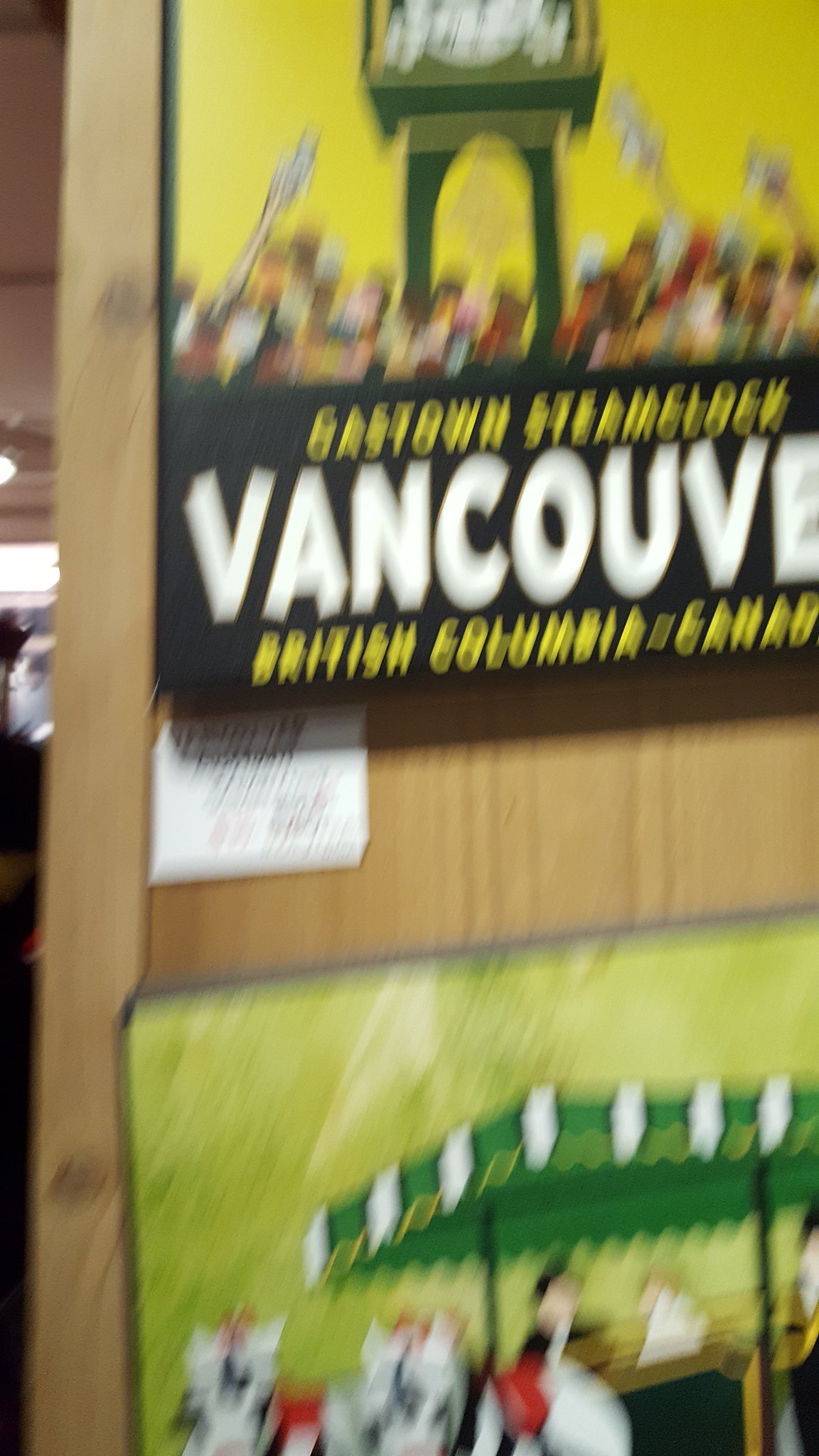The image depicts a somewhat blurry view of two tin posters displayed on a light brown wooden board, possibly for sale. The board is set against a backdrop that could either be a brown wall or a door, with a view of a room on the left-hand side. The top poster features a yellow sky background and a black clock tower labeled "Gaston Steam Clock" in Vancouver, British Columbia, Canada. The scene shows a crowd of people, distinguished by splotches of pink, red, yellow, and various shades of brown, pointing up at the clock. Below it, the second poster displays a green background with what seems to be a market stand. At the base of this image, it is difficult to identify clearly, but there appear to be zebras or horses. Some distinctive details, like a white tag with black and red text located between the posters, add to the overall composition, contributing to the slightly obscured but intriguing visual.